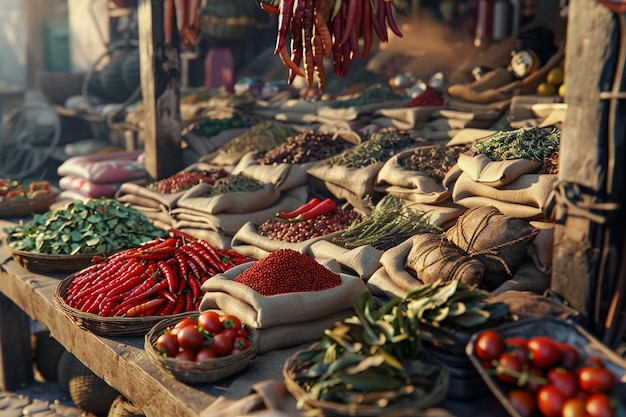This image captures a vibrant, rustic spice and vegetable market, likely in a culturally rich setting such as Latin America, the Middle East, or possibly India. The market exudes an old-world charm, with wooden shelves and tables displaying an abundant variety of fresh produce in burlap sacks and baskets. The front rows prominently feature vividly colored items like cherry tomatoes, green peppers, basil, and red chili peppers. Notably, the rustic wooden planks and folded burlap bags add to the market's primitive allure. Further back, additional sacks filled with an array of spices, herbs, and vegetables create a layered visual feast. Suspended above are strings of chili peppers, contributing to the market's dynamic and appealing atmosphere. Sunlight illuminates the scene, suggesting late afternoon or early evening, enhancing the market's vibrant, fresh, and inviting ambiance.